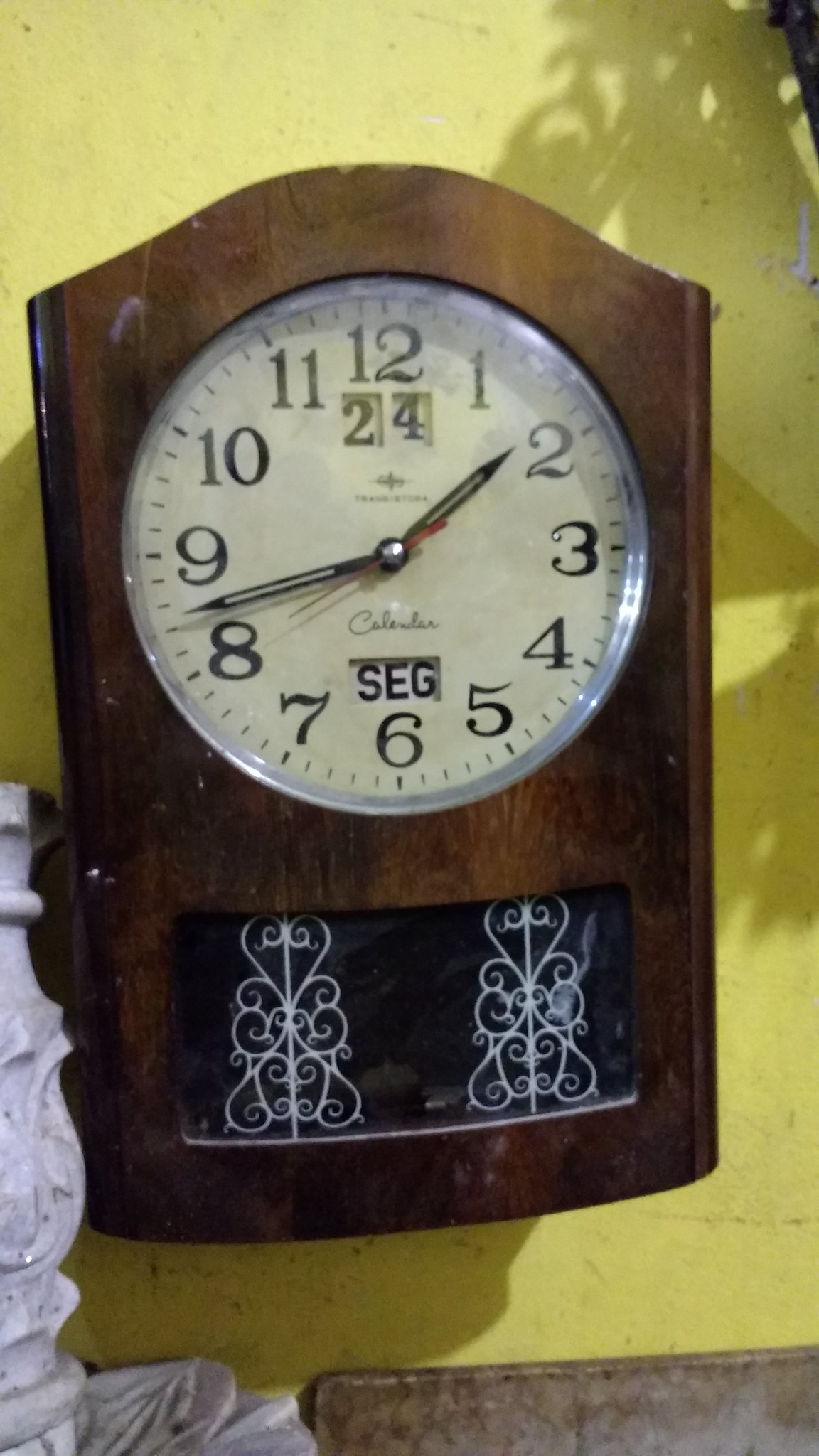This image features a detailed photograph of a wall-mounted clock set against a yellow stucco wall. The clock, encased in a wooden frame with both dark and light brown grains, has a roughly rectangular shape, with an arching bow at the top. The white clock face, protected by a glass cover, displays Arabic numerals from 1 to 12 in black. Below the number 12, two small windows show the date as the 24th. At the bottom of the clock face, above the number 6, a window displays the letters "S-E-G," likely indicating a day of the week in a foreign language, with the word "Calendar" written in cursive above it. The clock's hands include a black minute and hour hand with a white stripe and a pointed arrow, as well as a red second hand. Below the main clock face, the wooden case features two intricate plastic or wire designs. In the lower left corner, an ornate white stone vase or sculpture is partially visible, and at the bottom of the image, a thin strip of brown suggests a piece of furniture.